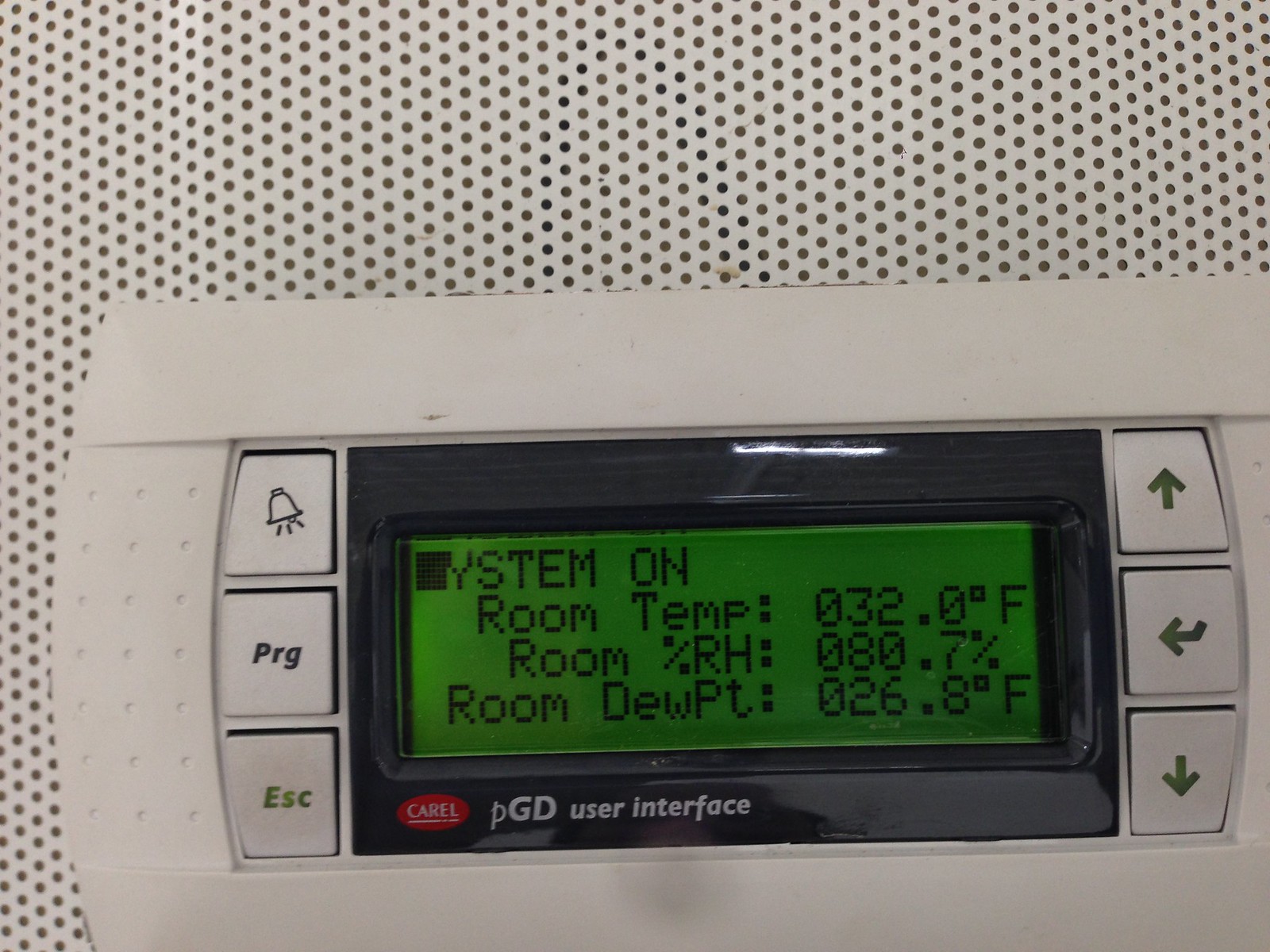A detailed close-up image of an older-model thermostat mounted on a wall. The wall features a unique design with numerous black dots arranged in a diagonal pattern. The thermostat itself is predominantly white and appears slightly dated. It is equipped with six buttons surrounding the green display screen: the top-left button has an alarm bell symbol, the middle-left button is labeled "PRG" for program, the bottom-left button is labeled "ESC" for escape, the top-right button has an up arrow, the middle-right button features an enter symbol, and the bottom-right button has a down arrow. 

The green screen displays various readings in black text. The words "system on" appear at the top, with the "S" replaced by a black box. Below that, it reads "Room Temp: 32.0°F", "Room %RH: 80.7%", and "Room Dewpoint: 26.8°F". At the bottom of the screen, the brand "CAREL" is displayed within a red oval, followed by "pGD User Interface" in uppercase and lowercase letters.